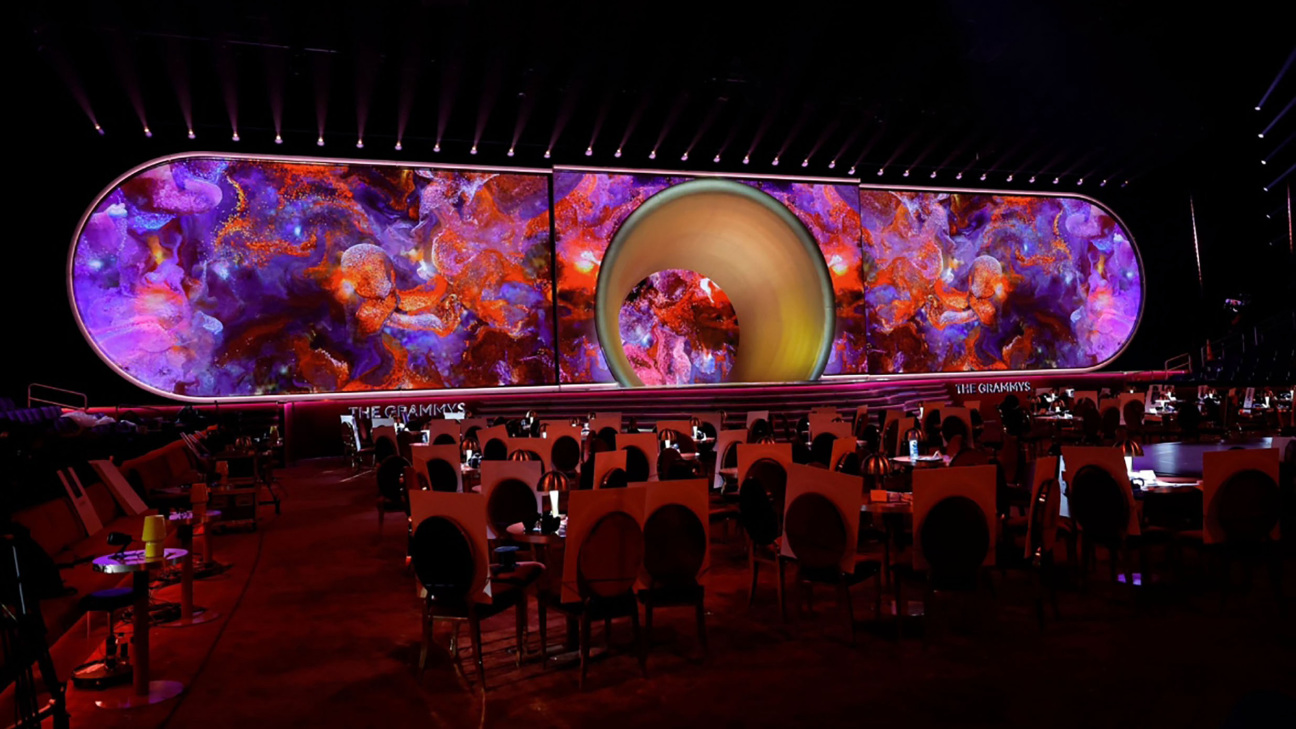This color photograph, in landscape orientation, captures an interior view of a grand concert hall prepared for the Grammys. The image prominently features a large stage adorned with a red carpet that extends onto the steps leading to it. The backdrop of the stage is dominated by a massive elliptical screen displaying an abstract, cosmic-like design with swirling patterns in shades of red, purple, and blue. In the center of this backdrop is a circular tunnel with a gold ceiling and walls, adding a touch of grandeur.

The stage spans the entire width of the photograph, and along the bottom edges, the text "THE GRAMMYS" is elegantly inscribed in silver metallic font. In front of the stage, there are multiple tables each accompanied by chairs, all set up with place cards indicating reserved seating for specific attendees. Candles are placed in the center of the tables, ready to be lit for the event. The seating area is on a single level, contributing to the expansive and unified look of the hall. The room is currently empty, with no guests seated yet, and is dimly lit to replicate the ambiance expected when the audience arrives. This detailed setup enhances the anticipation of a prestigious and visually captivating Grammy event.